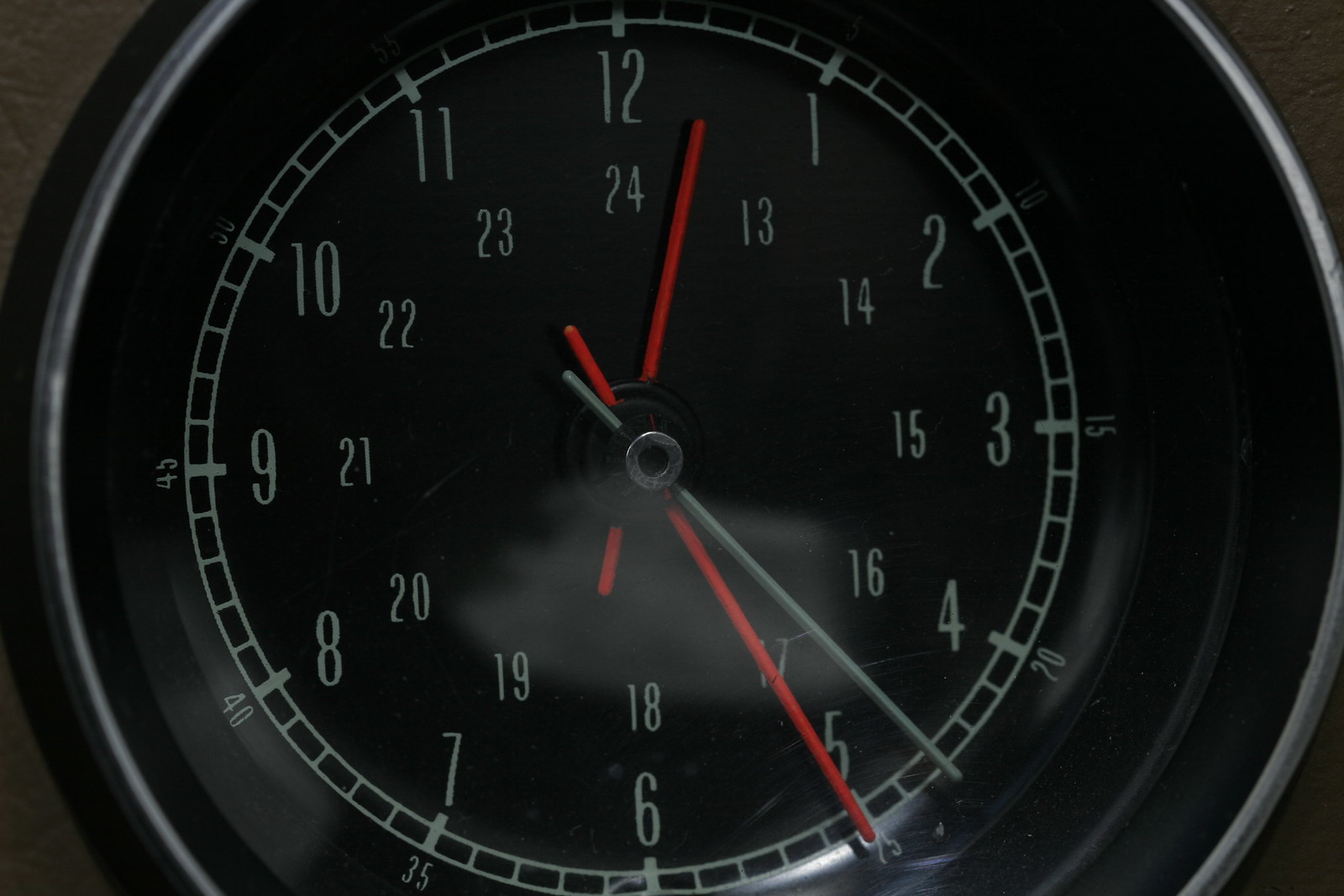The image is a close-up photograph of a round clock inset into an instrument panel, most likely inside a car, shown in landscape orientation. The exterior of the clock is silver while the dial itself is black. Surrounding the dial are two concentric green circles with smaller tick marks in between; some of these marks are heavier, aligning with the numbers. The clock features white text displaying hour numbers from 1 to 12, with additional inner markings showing 24-hour time, numbered from 13 to 24 beneath each corresponding hour. Every increment of five minutes around the outer edge is indicated by small square shapes. The clock has three hands: two red and one silver, all thin, used for indicating the time. The detailed marks and dual time readings suggest a precise, possibly automotive instrument.